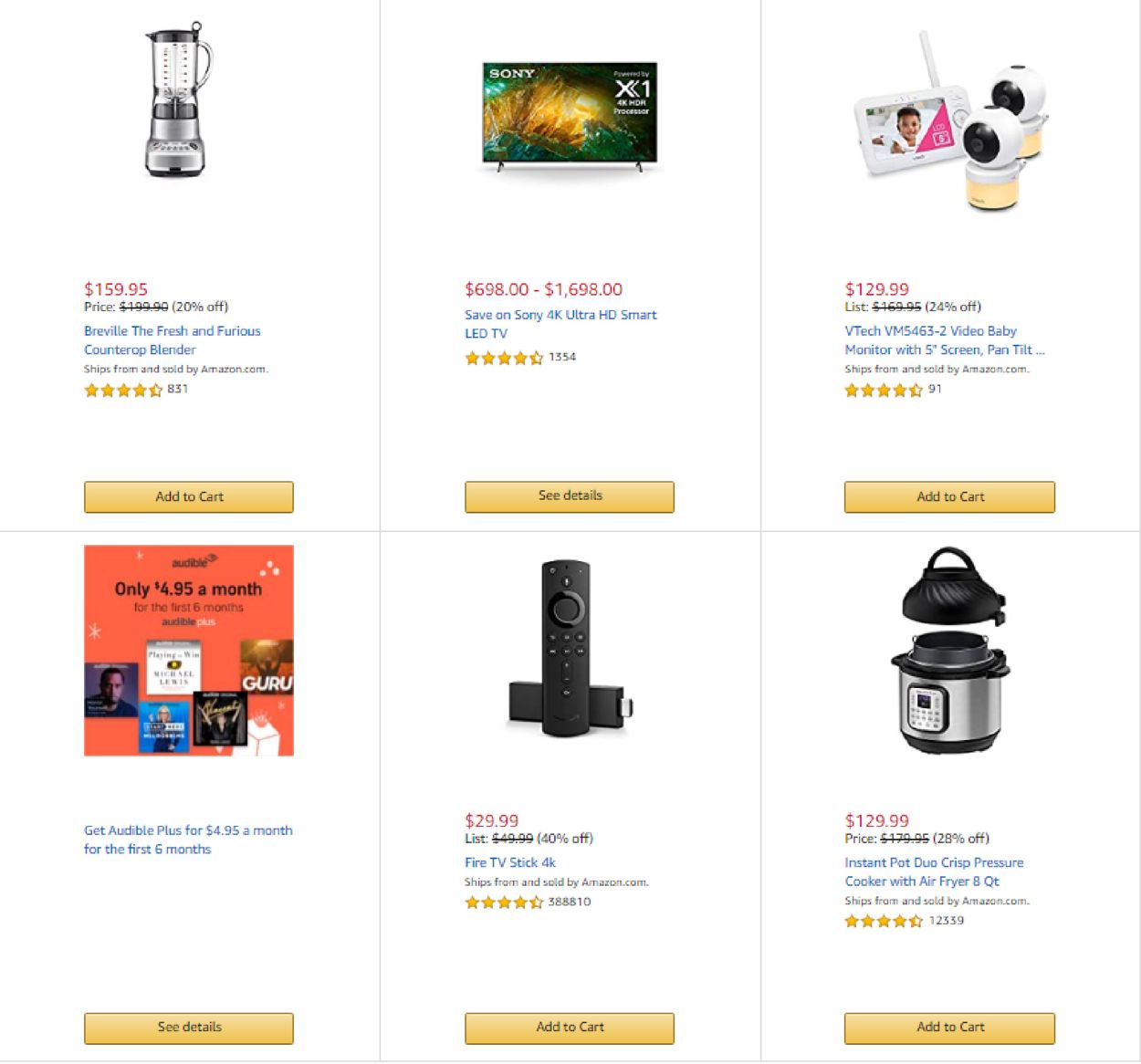The Amazon shopping cart displays a selection of six items, neatly organized over two rows:

1. **Item 1: Fresh and Furious Countertop Blender**
   - **Price:** $159.95 (20% off)
   - **Rating:** 4 stars
   - **Description:** A versatile countertop blender branded "Fresh and Furious."
   - **Add to Cart:** Available

2. **Item 2: Sony 4K Ultra HD Smart LED TV**
   - **Price:** $1,698.00 (save $698.00)
   - **Rating:** Not specified
   - **Description:** A high-definition Sony television featuring an image from a gym scene.
   - **Add to Cart:** Available

3. **Item 3: Baby Monitor with Two Cameras**
   - **Price:** Not specified
   - **Rating:** Not specified
   - **Description:** A baby monitor featuring a white screen, an image of a baby, and two round cameras.
   - **Add to Cart:** Available

4. **Item 4: Audible Plus Subscription Advertisement**
   - **Price:** $4.95 per month for the first six months
   - **Rating:** Not applicable
   - **Description:** Advertisement showcasing an Audible subscription featuring an assortment of book covers.
   - **Add to Cart:** Not applicable (subscription link available)

5. **Item 5: Fire TV Stick 4K**
   - **Price:** $29.99 (40% off)
   - **Rating:** 4 stars
   - **Description:** A compact media streaming device that plugs into your TV via USB, featuring a remote control.
   - **Add to Cart:** Available

6. **Item 6: Duo Crisp Pressure Cooker with Air Fryer (8QT)**
   - **Price:** $129.00 (28% off)
   - **Rating:** 4 stars
   - **Description:** A multifunctional pressure cooker and air fryer in silver with a black top.
   - **Add to Cart:** Available

This shopping cart offers a diverse range of items from kitchen appliances to electronics, each detailed with pricing and discount information as well as available actions.